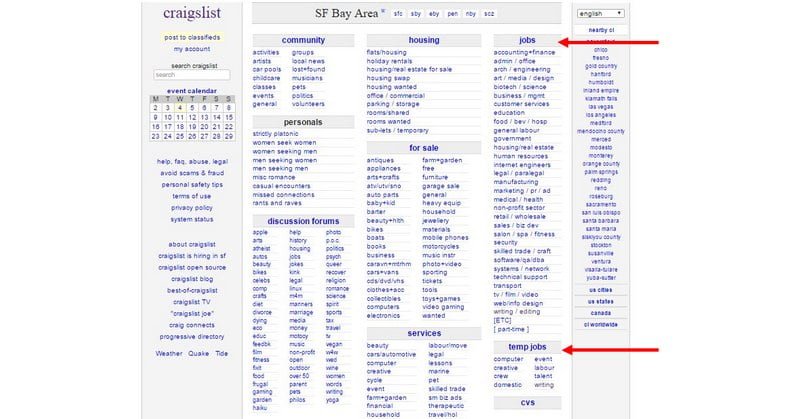Here we have a detailed snapshot of the Craigslist website, which was once immensely popular yet infamously associated with some dangers. The interface is predominantly gray and white. On the left side, the column showcases a purple-colored Craigslist logo. This column includes several functional links such as "post to classifieds," "my account," "search Craigslist," and an event calendar. It also provides essential links for "FAQ," "help," "abuse," "avoiding scams," among other informational resources.

Prominently in the center, the page identifies the local Craigslist area as San Francisco Bay Area. This section offers various major categories, including "community," "personals," "discussion forums," "services," "for sale," "housing," and "jobs." Each primary category further breaks down into a list of detailed subcategories, providing users with a comprehensive range of options to navigate through.

On the right side, there's a language drop-down box set to English by default, alongside options for selecting neighboring or related Craigslist locations within California. All these elements collectively create a multifaceted, user-friendly interface tailored to meet diverse user needs.